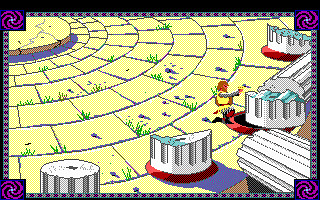This is a pixel art screenshot from a game, depicting a small, intricate scene. The focal point is a raised platform located in the top left corner, surrounded by an area constructed from increasingly larger bricks that converge towards the platform. In the scene, there is a figure dressed in a yellow outfit with arms outstretched, appearing to be kneeling. This figure is positioned among the remains of what were once Roman pillars; only the bases are intact, with the tops of two pillars visibly broken off and lying nearby. The ground, made of cement, has grass sprouting through its cracks, adding a sense of decay and nature reclaiming the space. The entire image is framed by a pixelated white and purpley border, featuring black hole-like swirls in each corner, composed of purple spirals, enhancing the mystical and aged atmosphere of the artwork.